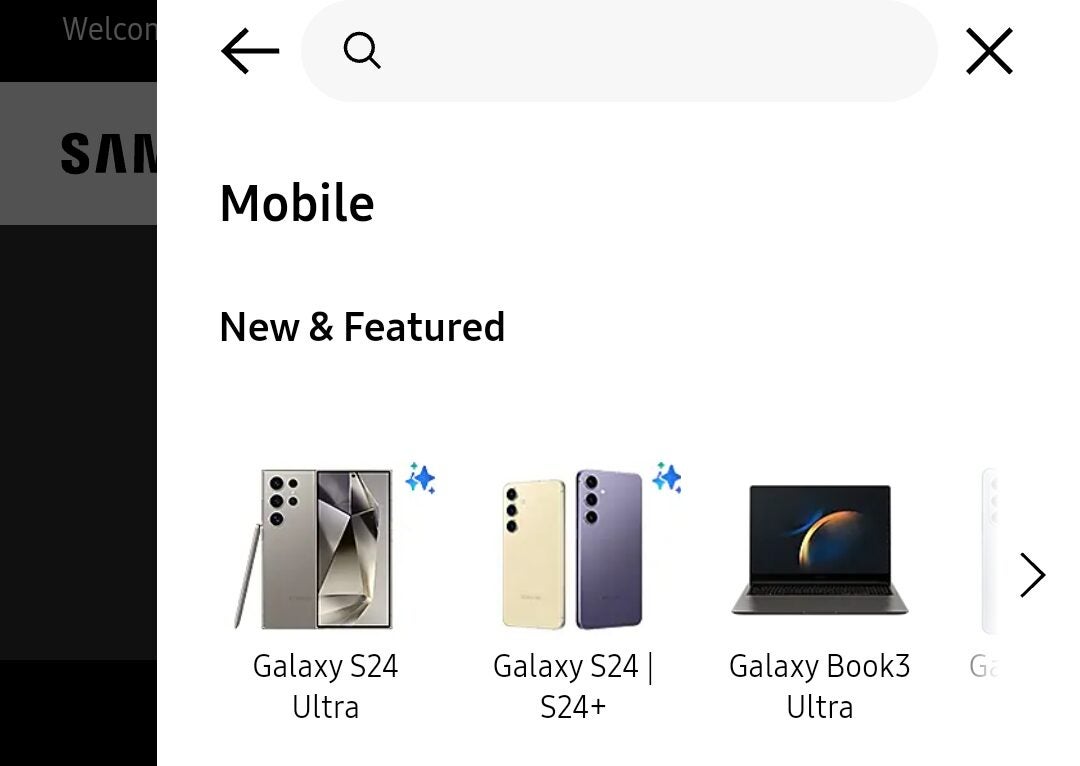This screenshot, in landscape orientation, captures a pop-up overlay on a mobile device's screen, likely from a Samsung shopping site. In the background, one can faintly discern elements of a mobile phone message interface. The foreground comprises a rectangular pop-up window set against a two-column layout. 

The left column is a black vertical stripe extending from the top left to the bottom left of the image. Near the upper part of this stripe, "Samsung" is partially visible, with the letters "S-A-M" prominently displayed. A white stripe overlays part of the black column, inscribed with the word "Welcome."

The main focus is the pop-up message, a prominent white block taking up most of the right column. The top row of this pop-up includes a back button, a search bar, and an "X" icon for closing the window, all set against a black background. Beneath this row, bold text reads "Mobile," followed by another line of bold text stating "New and featured."

Displayed prominently in the pop-up are three Samsung products: the Galaxy S24 Ultra, the Galaxy S24/S24 Plus, and the Galaxy Book 3 Ultra. At the bottom right corner of the image, there is a "G" symbol and a right-pointing arrow, suggesting a navigation button for more options.

The overall impression is that this is a promotional interface from a Samsung shopping site, showcasing their latest products. Clicking on any of the listed items likely redirects users to detailed product pages, possibly allowing for direct purchase options.